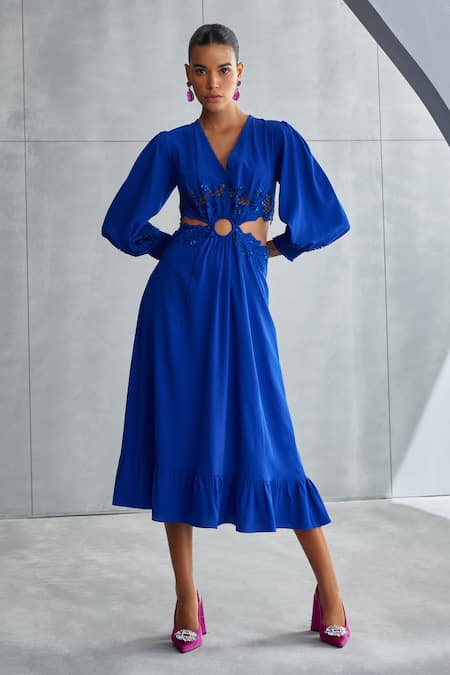This photograph captures a woman of presumed Hispanic descent posing in a stylish dark blue dress. Her hair is black, tied back slickly, and she has medium to dark skin. The dress is intricately designed with baggy, long sleeves and extends down from the midsection to well below her knees, featuring unique openings: three distinct slits that reveal parts of her skin — one central revealing her stomach and two additional slits on either side. Her accessories include pink to purple earrings and matching high heels adorned with a single white flower on each toe. The model’s pose is confident, with one hip slightly cocked and her hands positioned behind her back at her waist. She stands against a background of large concrete tiles with a hint of a blue pattern emerging from the top right corner, potentially a gray office building, with a touch of sunlight illuminating the right side.